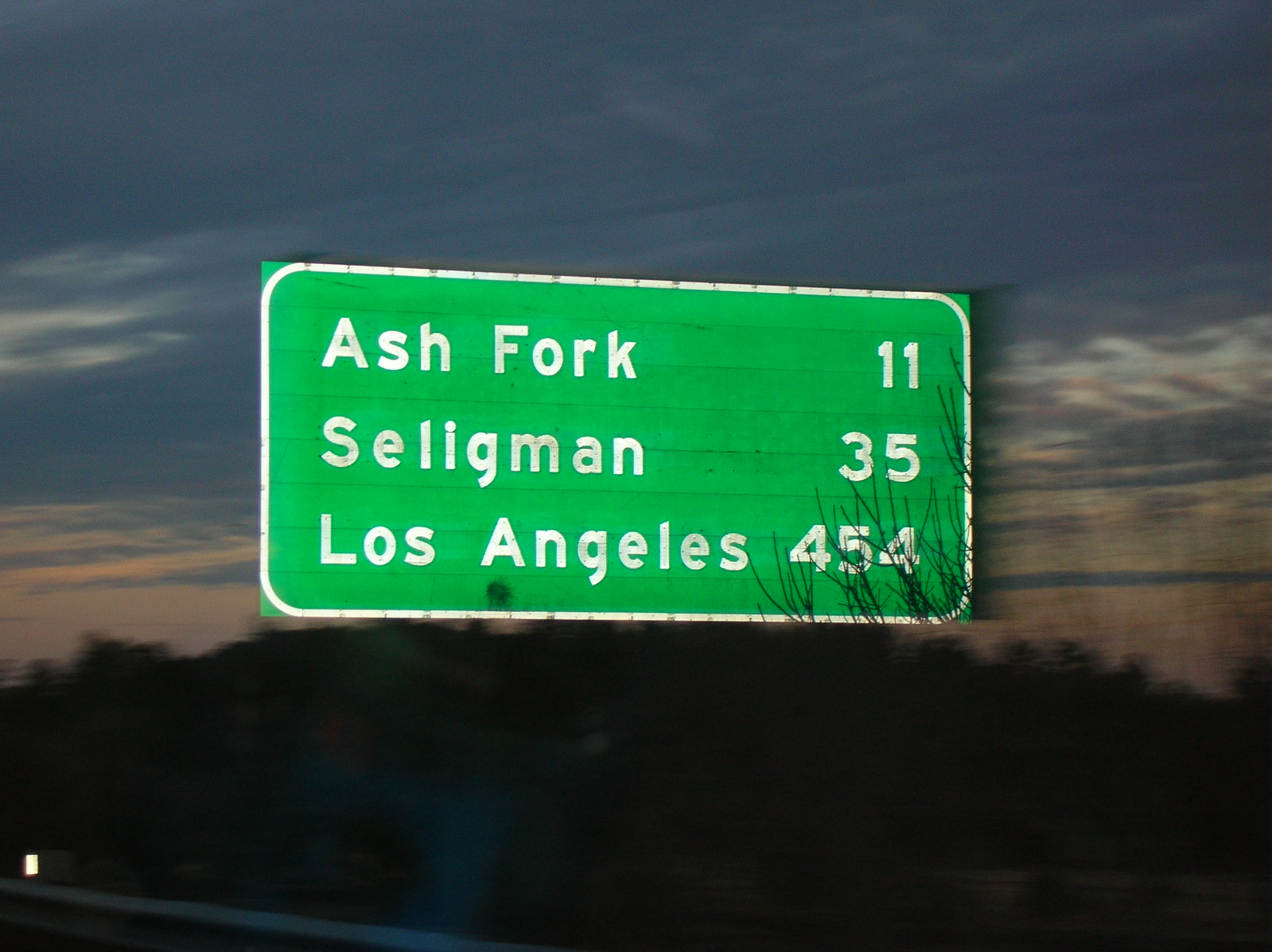In this photo taken just after sunset, we see a large rectangular green mileage sign with a white border and white lettering that reads from top to bottom: Ash Fork, 11 miles; Seligman, 35 miles; and Los Angeles, 454 miles. The numbers 454 and parts of the 35 and 11 are slightly obscured by overhanging branches. The sky above the sign transitions from a darker blue with a faint brownish haze just above the trees to a softer hue with dark, low-lying clouds. A touch of pink is evident, suggesting the sun has just set. Headlights likely illuminate the sign, casting a slight reflection, possibly from a vehicle's windshield. The surroundings include a gray road railing at the bottom left and a backdrop of blurry green trees that appear almost black due to the low light.